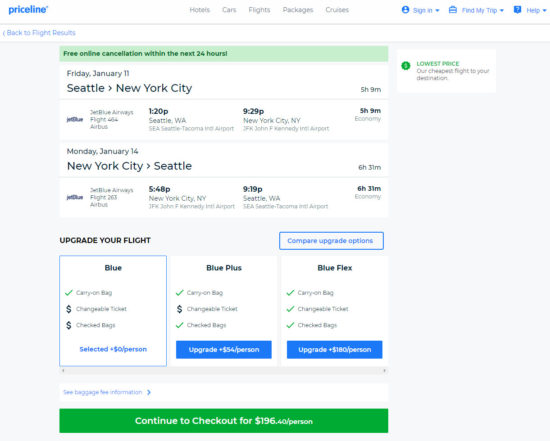Screenshot of a Priceline.com webpage displaying flight options. The top menu features clickable tabs in gray for "Tickets," "Cars," "Flights," "Packages," and "Cruises," with blue options for "Sign In," "Find My Trip," and "Help." Below, a link labeled "Back to Flight Results" is visible.

The main section highlights a flight from Seattle to New York City scheduled for Friday, January 11th, with a policy of free online cancellation within the next 24 hours. The flight, covered by a lowest price guarantee, details a departure from Seattle at 1:20 PM, arriving in New York City at 9:29 PM. This is an economy class flight, and an additional returning flight from New York City to Seattle is available for Monday, January 14th, departing at 5:48 PM and arriving at 9:19 PM, with a total duration of six hours and three minutes.

There are options to upgrade the flight experience with Blue, Blue Plus, or Blue Flex packages. The total cost for this itinerary is $196, with a prompt to "Continue to Checkout" prominently displayed.